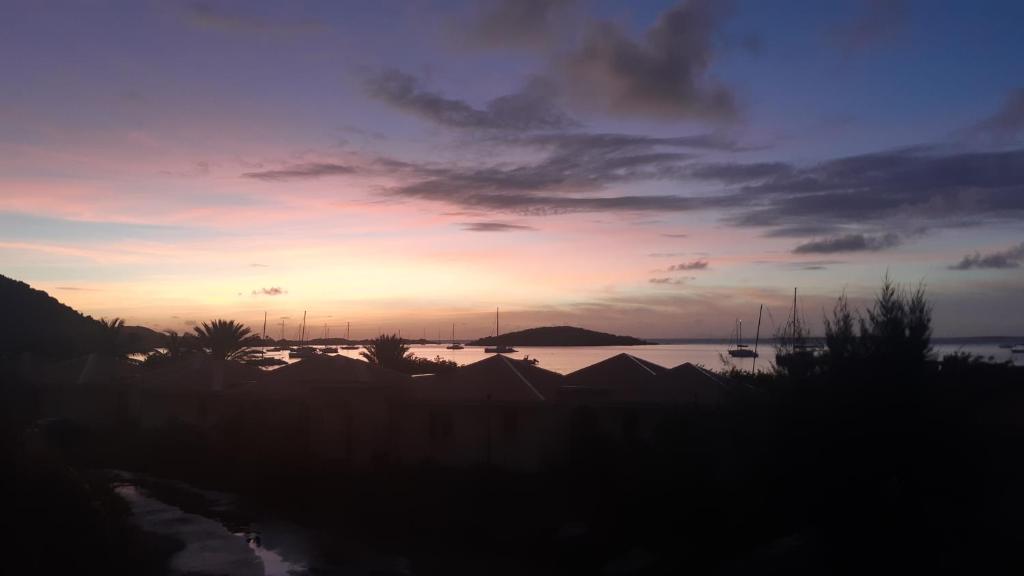The image captures a dimly lit scene, likely during either sunrise or sunset, with emphasis on the sky's subtle hues. The sky features a gradient of colors, transitioning from hints of yellow, pink, and orange to patches of dark blue and gray clouds. Beneath this colorful display, the landscape is shrouded in darkness, rendering much of the foreground nearly indistinguishable. Silhouettes of trees border a still body of water, which takes up the central portion of the photo. At least a handful of boats are visible on the water's surface, and a landmass, including a hill structure on the left, extends across the frame. There are indications of houses and a puddle in what seems to be a very dark lower portion of the image, reinforcing the underexposed nature of the photograph. The overall scene is quiet and serene, evoking a tranquil atmosphere amidst the low light.